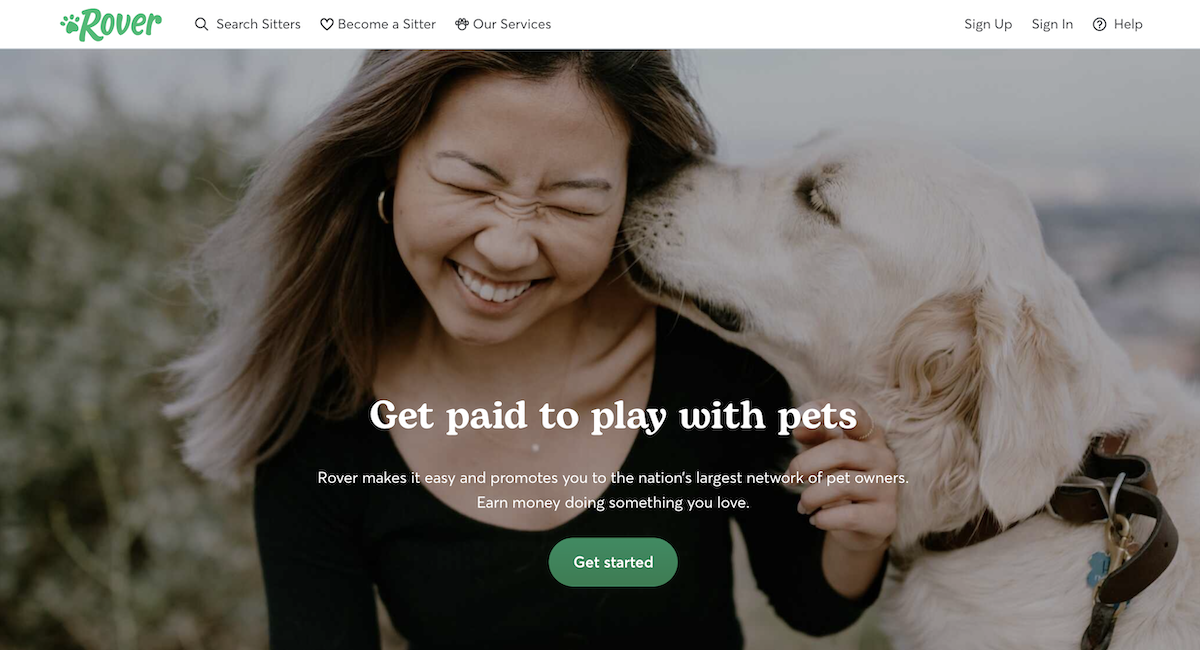The image features the homepage of the Rover website, a platform dedicated to connecting dog owners with pet sitters. The top of the page prominently displays the Rover logo in green, accompanied by a small dog paw print. Navigation options include "Search Sitters," "Become a Sitter," "Our Services," as well as "Sign Up," "Sign In," and "Help" buttons for further assistance.

At the center of the page, a bold message invites users to "Get paid to play with pets," emphasizing how Rover simplifies the process and connects sitters with the nation's largest network of pet owners. Below this message, a green "Get Started" button encourages immediate action.

The central image showcases an Asian woman being affectionately licked by a small white Labrador. The woman, dressed in a long-sleeve black shirt, appears to enjoy the playful interaction despite her hand being up in a playful attempt to shield herself. Her face is scrunched up with a smile, and her teeth are visible as she squints from the dog's nuzzling on her ear. The dog also wears a black collar and has a tuft of fur under his left ear. The background suggests an outdoor setting, with glimpses of trees and possibly water.

In summary, the website offers two main services: finding a dog sitter or becoming one, aiming to provide detailed information and easy navigation for pet owners and potential sitters alike.